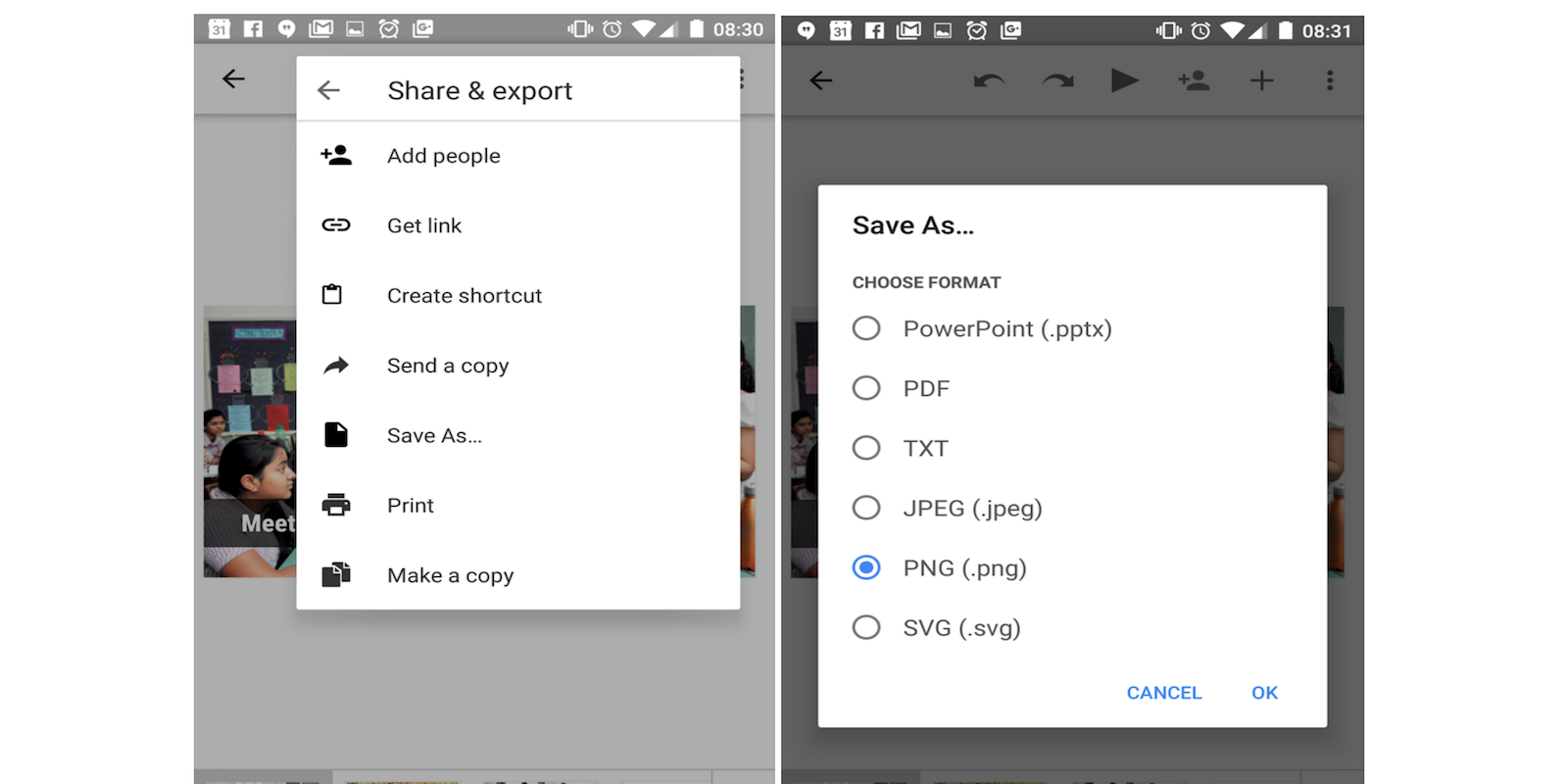The image shows two smartphone screens side by side, each displaying different menu options in a white rectangular pop-up. 

The left screen displays a menu titled “Share and export” with an arrow pointing to the left. Below the title, there are several icons listed vertically with corresponding actions:
1. A plus symbol followed by the text “Add people.”
2. A paperclip with the text “Get link.”
3. A box symbol with the text “Create shortcut.”
4. An arrow pointing to the right with the text “Send a copy.”
5. An icon resembling a piece of paper with a corner folded down and the text “Save as...”
6. A printer icon with the text “Print.”
7. An icon with two overlapping pieces of paper and the text “Make a copy.”

The right screen focuses on a specific action from the "Save as..." menu. At the top, the text reads “Save as...” followed by “Choose format.” Below this title, there are six circular icons aligned on the left, each representing a different file format. Next to each icon, the corresponding file format is listed:
1. PowerPoint
2. PDF
3. TXT
4. JPEG
5. PNG (highlighted or selected)
6. SVG

The selected option, PNG, indicates that the user has chosen to save the file in the PNG format.